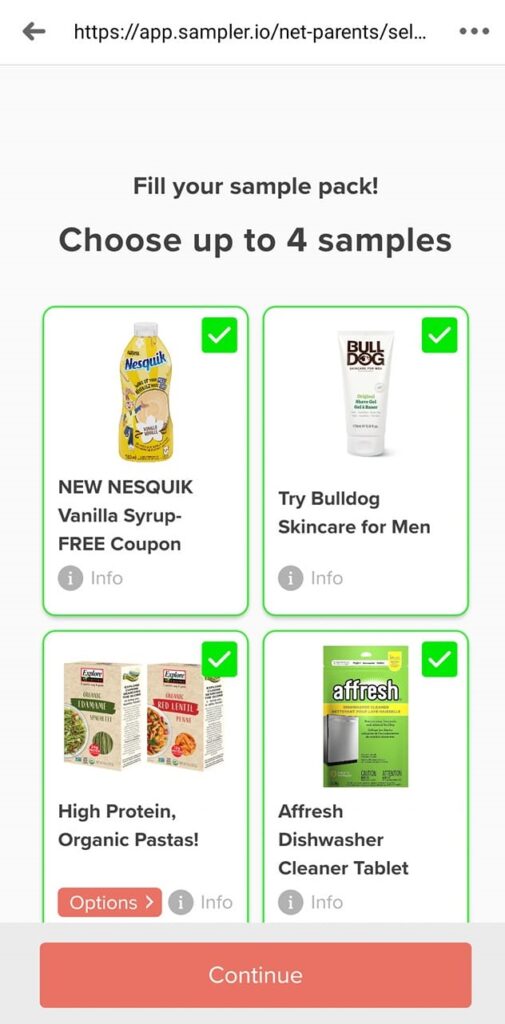**Detailed Caption:**

The image is a screenshot taken from a smartphone showcasing a webpage at the URL "https://app.sampler.io/net-parents/SEL." At the top of the screen, there is a back arrow icon pointing to the left, followed by the URL. To the right, there are three vertical black dots indicating a menu or additional options.

Below this, there is a gray section with the text "Fill your sample pack, choose up to four samples." The screen displays that the user has selected four samples, each inside a distinct gray rectangle. 

1. On the upper left is the first sample, labeled "New Nesquik Vanilla Syrup Free Coupon." There is an image of a yellow bottle with "Nesquik" written on it. A confirmation green square with a white checkmark is located in the upper right corner of this sample box.

2. To the right is the sample for "Try Bulldog Skincare for Men," which includes an image of a white bottle labeled "Bulldog" in blue text. There is a similar green square with a white checkmark in the upper right corner, indicating selection.

3. On the bottom left, the sample is "High Protein Organic Pasta," with an accompanying orange "Options" button beneath the text. The sample box also features a green square with a white checkmark in its upper right corner.

4. Lastly, to the right of the pasta sample, there is a sample for "Affresh Dishwasher Cleaner Tablet." The packaging is green and labeled "Affresh." This sample too has a green confirmation square with a white checkmark in the upper right corner.

At the very bottom of the screen, an orange "Continue" button is visible, allowing the user to proceed further in the process.